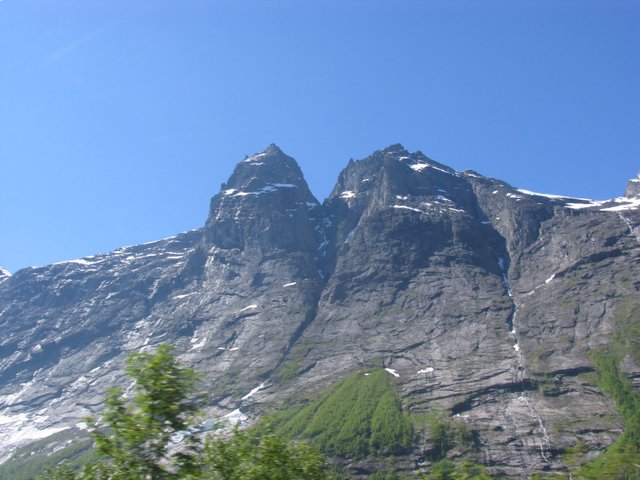The image showcases a majestic, steep mountainside characterized by predominantly black and dark gray rocky terrain. The mountain, which extends vertically in a wide, rectangular frame, is adorned with patches of white snow scattered across its rugged surface, more pronounced along the top ridges. At the base of this imposing cliff face, pockets of vibrant greenery emerge, including clusters of green leaves and possibly moss-like growth, particularly towards the bottom right and center of the image. The scene is framed by a clear blue sky, contrasting sharply with the stark, rocky peak that juts upward in two circular mounds forming a small V-shape in the middle. Additionally, the lower parts of the image feature treetops, predominantly on the left side, where a few deciduous trees can be spotted. Together, these elements create a visually striking composition that captures the raw beauty and varied textures of the mountain landscape.